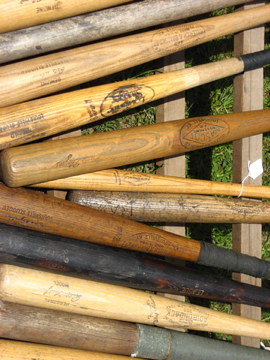This image captures a close-up, bird's-eye view of a collection of vintage and antique wooden baseball bats laid out on a bench with grass visible underneath. The bats, numbering at least 11 with a partial view of a 12th, display a range of colors and significant wear, indicating extensive use over the years. Their hues vary from light browns and tan to darker browns, with one bat notably painted black. Several of the bats feature tape around their handles, with grey tape being prominent on one of the darker bats. Despite the age-related wear and scratches, faint inscriptions are visible on about half of the bats, though none are legible. The backdrop includes brown 2x4 wooden structure elements and green foliage peeking through, further enhancing the rustic and nostalgic appeal of the scene.